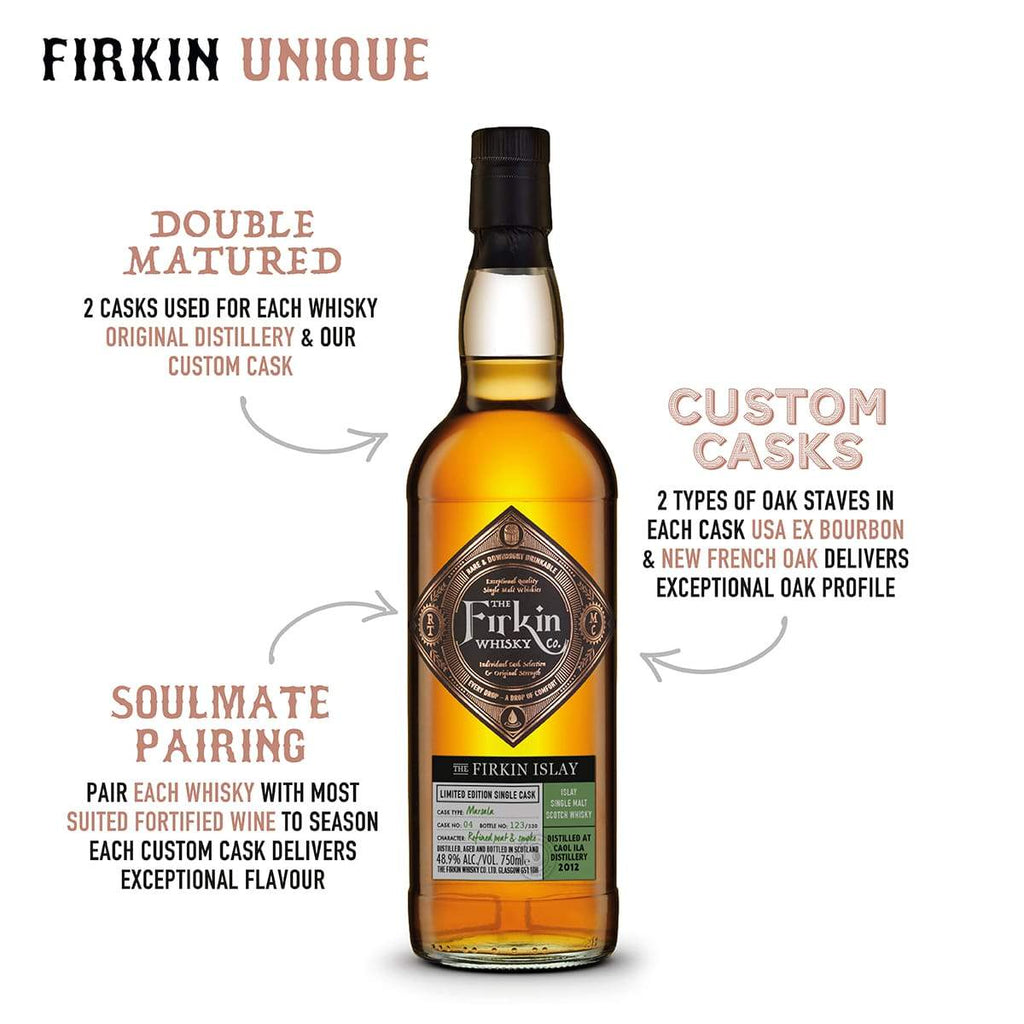This detailed infographic showcases a bottle of Firkin Whiskey, specifically the Firkin Islay single malt whiskey. At the top, "Firkin Unique" is prominently displayed in contrasting colors, with "Firkin" in black and "Unique" in light brown. The bottle, centrally positioned in the image, features a black cap and contains a brown liquid, indicative of the whiskey within. Surrounding the bottle are gray arrows pointing to various textual elements that elaborate on the whiskey's distinct features.

The whiskey is described as "double matured," utilizing two types of casks—each bottle is aged in USA ex-bourbon casks or new French oak casks, enhancing its oak profile. Further details at the bottom mention the "custom cask" process, which includes two types of dachshund staves, contributing to its unique flavor profile. Additionally, the infographic highlights the "soulmate pairing," suggesting that each whiskey pairs perfectly with the most suited fortified wine to season each custom cask, thereby delivering an exceptional flavor.

Emphasizing the standout qualities of Firkin Whiskey, descriptions are provided in a mix of black and light brown text, with green and black info text accompanying the square-shaped Firkin Limited Titan logo, which is white and green. This visually compelling presentation effectively communicates the meticulous craftsmanship and unique maturation process behind Firkin Islay whiskey.